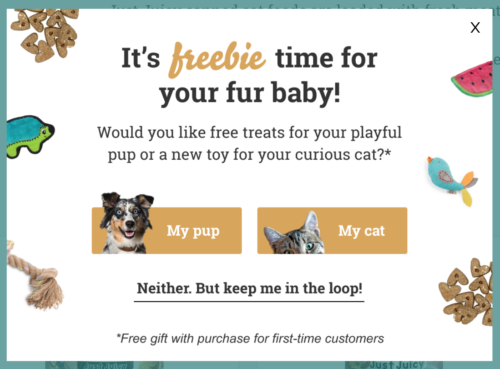In this image, we can see a prominently displayed "X" icon in the top right corner. The background is white, and the entire image is framed by a greenish-blue border. In the top left and bottom right corners, there are light brown heart-shaped dog food pieces, each featuring a small brown heart in the center.

At the top center of the image, the text reads, "It's freebie time for your fur baby." The word "freebie" is highlighted in an orangish cursive font. Below this, the text continues with the question, "Would you like free treats for your playful pup or a new toy for your curious cat?"

The image then splits into two categories: "My pup" on the left, accompanied by a picture of a dog, and "My cat" on the right, accompanied by a picture of a cat. Below these, a third option reads, "Neither but keep me in the loop," underlined with a black line.

At the very bottom center of the image, the text states, "Free gift with purchase for first time customers," marked by an asterisk to the left of the sentence.